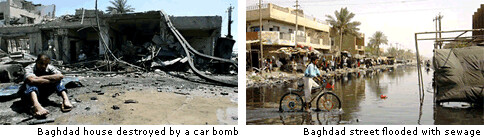The image consists of two side-by-side photographs, each with a descriptive caption underneath on a white background. The photograph on the left, labeled "Baghdad house destroyed by a car bomb," depicts a bombed-out, one-story concrete building with its front facade cratered and reduced to rubble. In the bottom left corner, a sorrowful man with dark hair, wearing a tan shirt and rolled-up denim jeans, sits on the ground with his arms folded over his knees and head bowed. The scene is lit by daylight, and other individuals can be seen amidst the debris inside what's left of the structure.

The photograph on the right, captioned "Baghdad street flooded with sewage," shows a street submerged in filthy water, resembling a river. The water level reaches halfway up the wheels of a blue-shirted cyclist seen riding from left to right. The background includes a two-story building on the left side, with piles of trash along what would be the sidewalk, and a truck moving through the floodwaters. The sky appears white, making the grim scene of a waterlogged, trash-lined street even more stark.